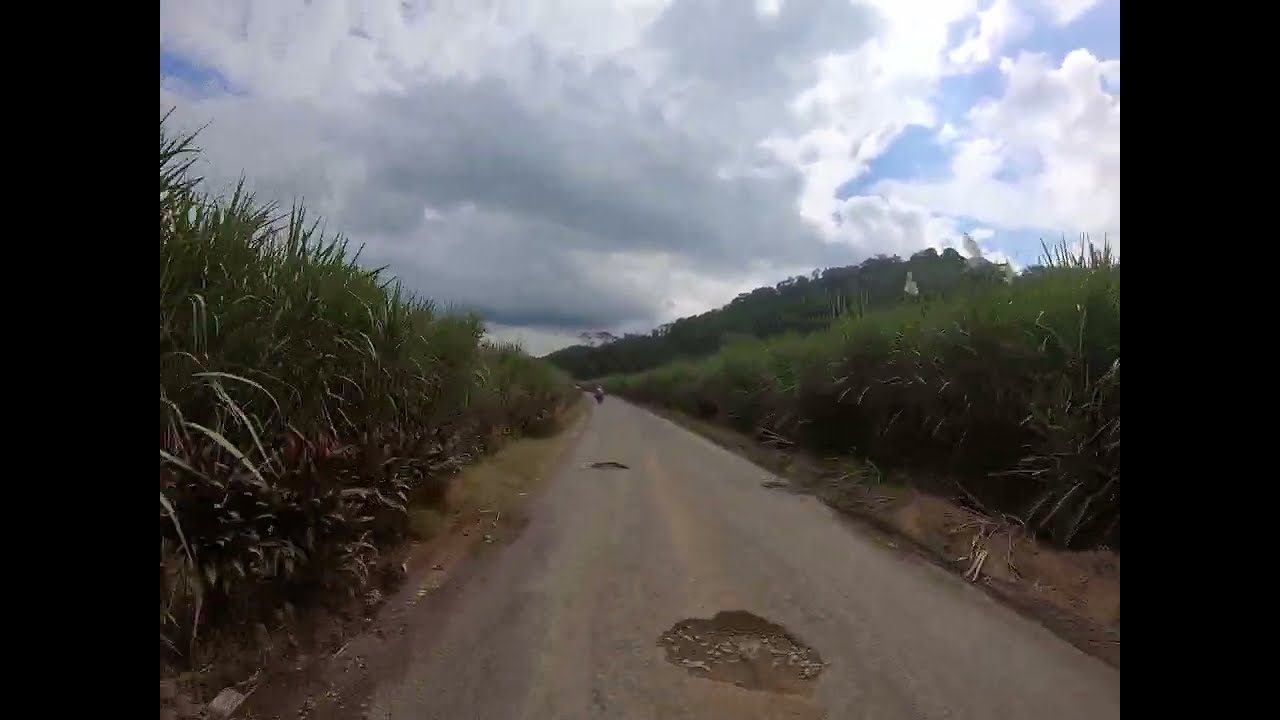The image is a detailed color photograph, taken in landscape orientation, likely as a freeze frame from a GoPro video mounted on a bike or scooter. The layout is framed by vertical black stripes on both the left and right sides. The main focus is a narrow, paved road that appears to be in a tropical setting, possibly resembling Puerto Rico or Hawaii, surrounded by dense, tall, dark green vegetation including spiky plants in the foreground.

The road itself is characterized by noticeable wear, featuring a series of potholes: a large one directly in front of the viewer, and two additional smaller potholes approximately 20 yards ahead, positioned left and right. Further down, the road gently curves to the left, where a motorcyclist is seen riding away in the distance. The backdrop includes gently rising hills to the right, adorned with trees. Overhead, a partly cloudy sky showcases puffy white and gray clouds with sunlight streaming through, adding a realistic, vibrant feel to the scene.